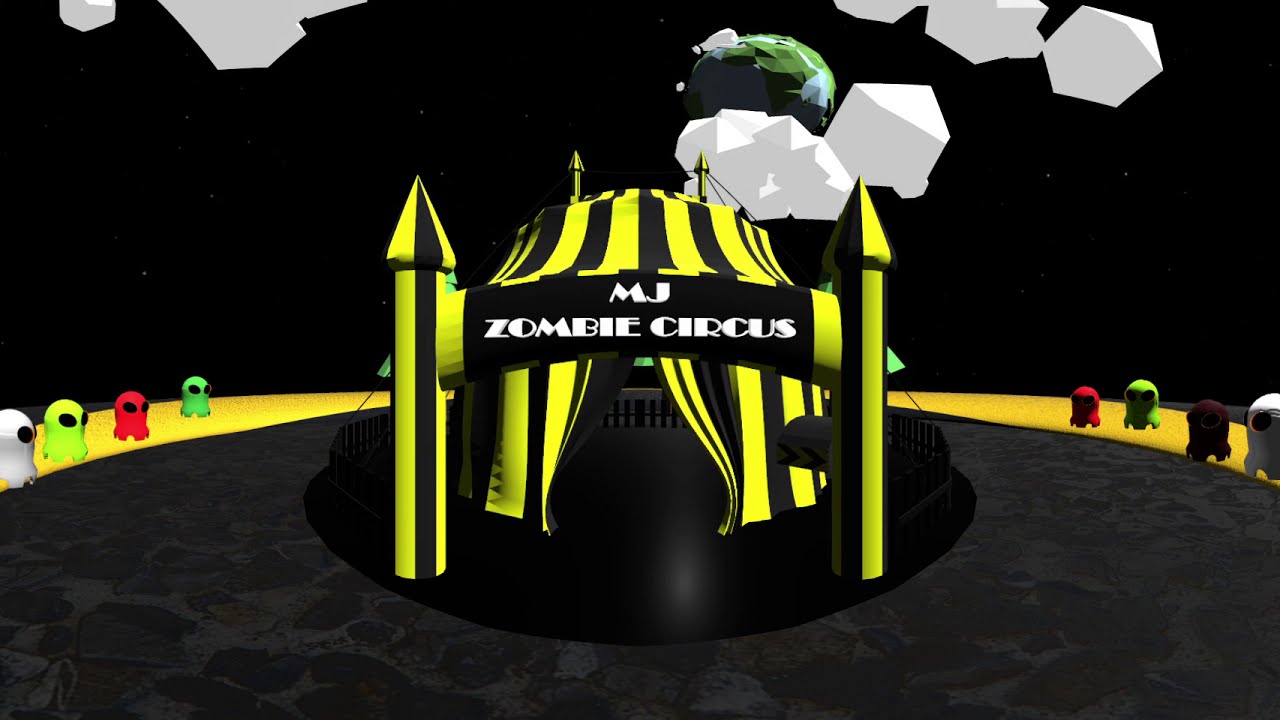The image is an animated 3D graphic resembling a circus scene titled "MJ Zombie Circus". Central to the image is a vertically striped, yellow and black circus tent with the text "MJ Zombie Circus" in white font on its facade. The tent is situated on a round black platform and is partially open, revealing a black picket fence behind it. The backdrop is a pitch-black sky scattered with white specks, likely representing stars, and features pixelated clouds and a heavily pixelated globe that appears to be Earth.

On either side of the platform, there are various small, ghost-like alien creatures in colors including white, green, red, purple, and a darker red. These creatures have alien-like faces or black eyes with flowing robes. Additionally, there are white, stone-like objects suspended in the air, adding to the surreal atmosphere of the scene.